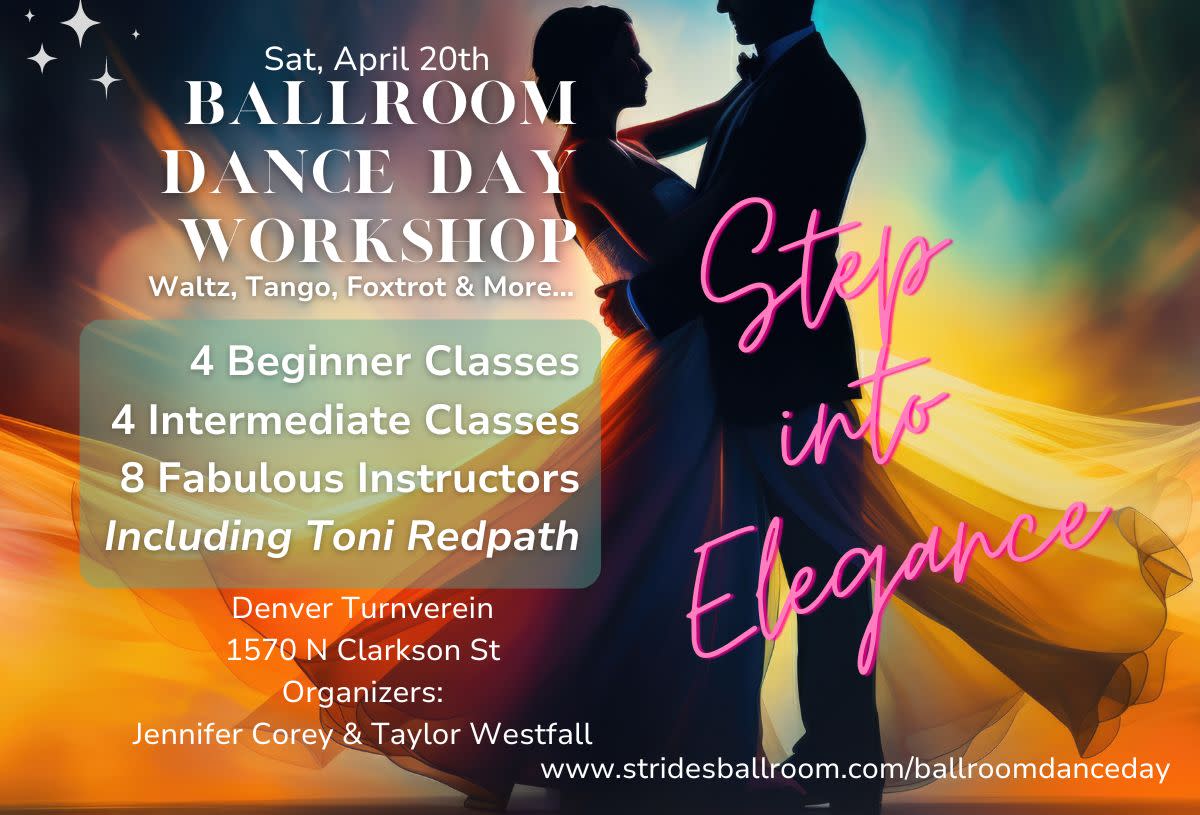Join us for the Ballroom Dance Day Workshop on Saturday, April 20th! This vibrant advertisement features a mid-dance couple clothed in formal attire—the woman in a partially transparent, flowing dress wrapped gracefully around her male partner, who wears a sleek tuxedo. Set against a backdrop of vivid blues, yellows, and pinks, their elegant movements evoke a sense of romance and sophistication. The text on the left announces a day filled with waltz, tango, foxtrot, and more, with four beginner classes, four intermediate classes, and eight fabulous instructors, including Tony Redpath. The venue is Denver Turnverein, located at 1570 North Clarkson Street. Organized by Jennifer Corey and Taylor Westfall, this event invites you to "Step into Elegance" in pink cursive, adorned with little diamond stars at the top left. For more details, visit www.stridesballroom.com/ballroomdanceday.